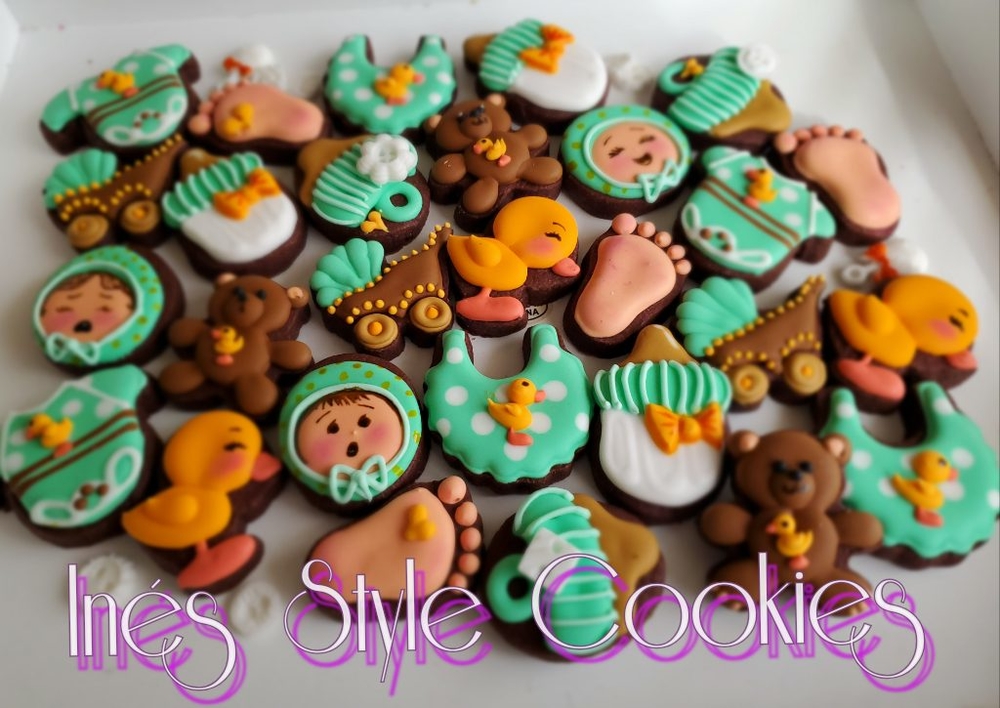This is an image showcasing an array of intricately decorated baby-themed cookies. They are set on a light gray background, and at the bottom, the text "Inez Style Cookies" is written in a special graphic style, indicating the brand name. The cookies come in various shapes and sizes, notably featuring designs such as yellow ducklings with orange beaks and feet, teddy bears with yellow ducks on their chests, baby faces wearing bonnets, baby bibs, and strollers. There are also cookies shaped like baby feet with detailed toes. Most of the cookies are brown, likely chocolate or gingerbread, and they're decorated with vibrant colors, primarily green, yellow, and accents of brown and gold. The photograph is high-quality, possibly showing the cookies inside an open box with light illuminating them. The overall theme is clearly aimed at celebrating newborns, with each cookie meticulously crafted to suit the occasion.